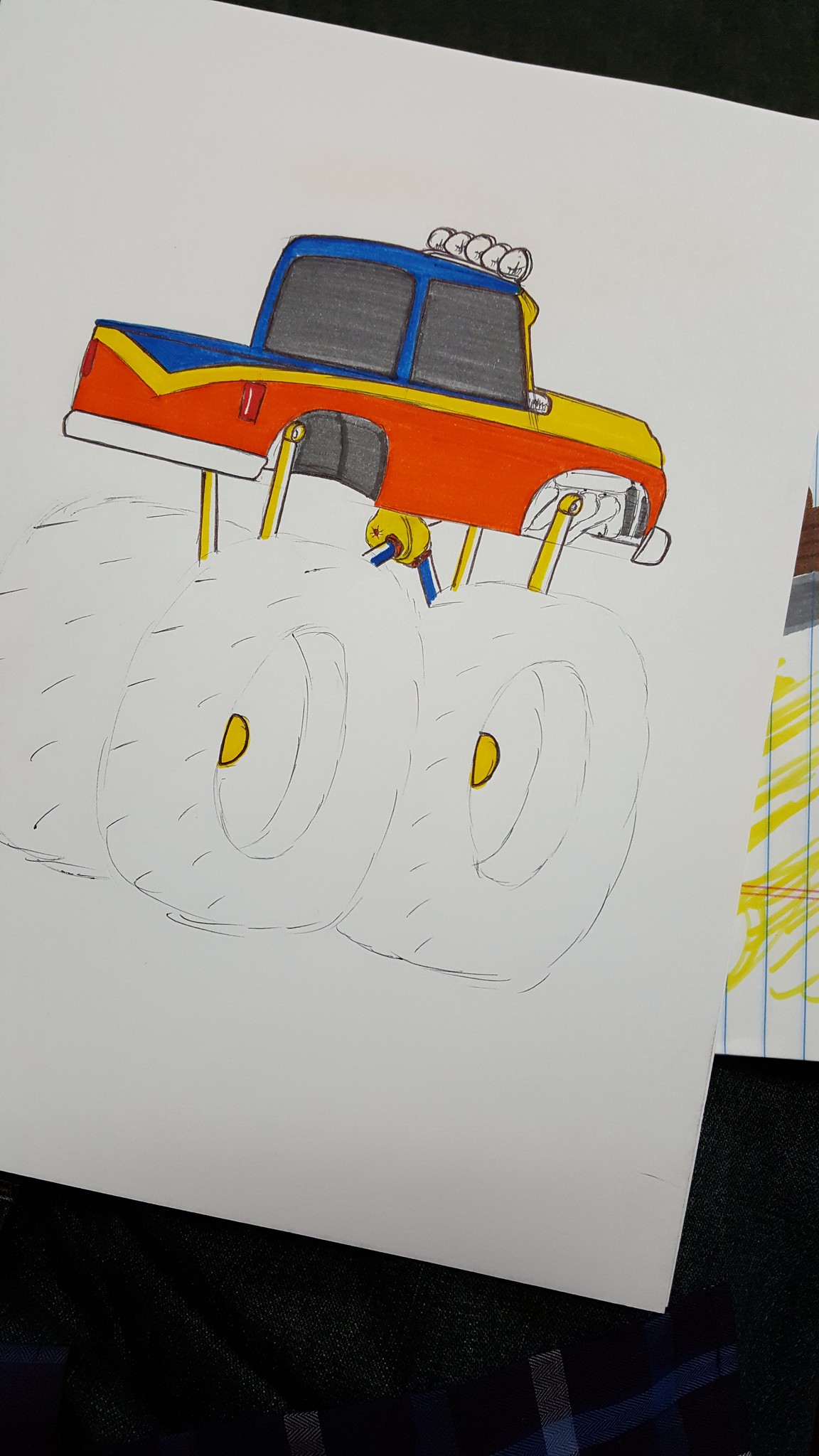This is a detailed and colorful child's drawing of a large monster truck on a white sheet of paper. The truck is painted in vibrant shades of blue, yellow, and red. A striking feature of the truck is its five large headlights positioned on the front of the roof. The truck sits high on its suspension, which comprises yellow shocks and seemingly blue leaf springs, partially obscured by the massive, outlined tires. The tires themselves are only penciled in without any color, creating a contrast with the rest of the drawing. The wheels have a distinctive yellow gold center that matches the truck’s overall color scheme. Additionally, the drawing includes dark-tinted windows. Surrounding the drawing are other elements – notably, a piece of notebook paper with blue and red guidelines and some brown, gray, and yellow scribbles, visible off to the right side of the image. At the bottom right and bottom center of the picture, a piece of fabric with blue and white stripes is also visible. Although still unfinished, the detailed rendering of the monster truck showcases the child's impressive use of color and attention to detail.